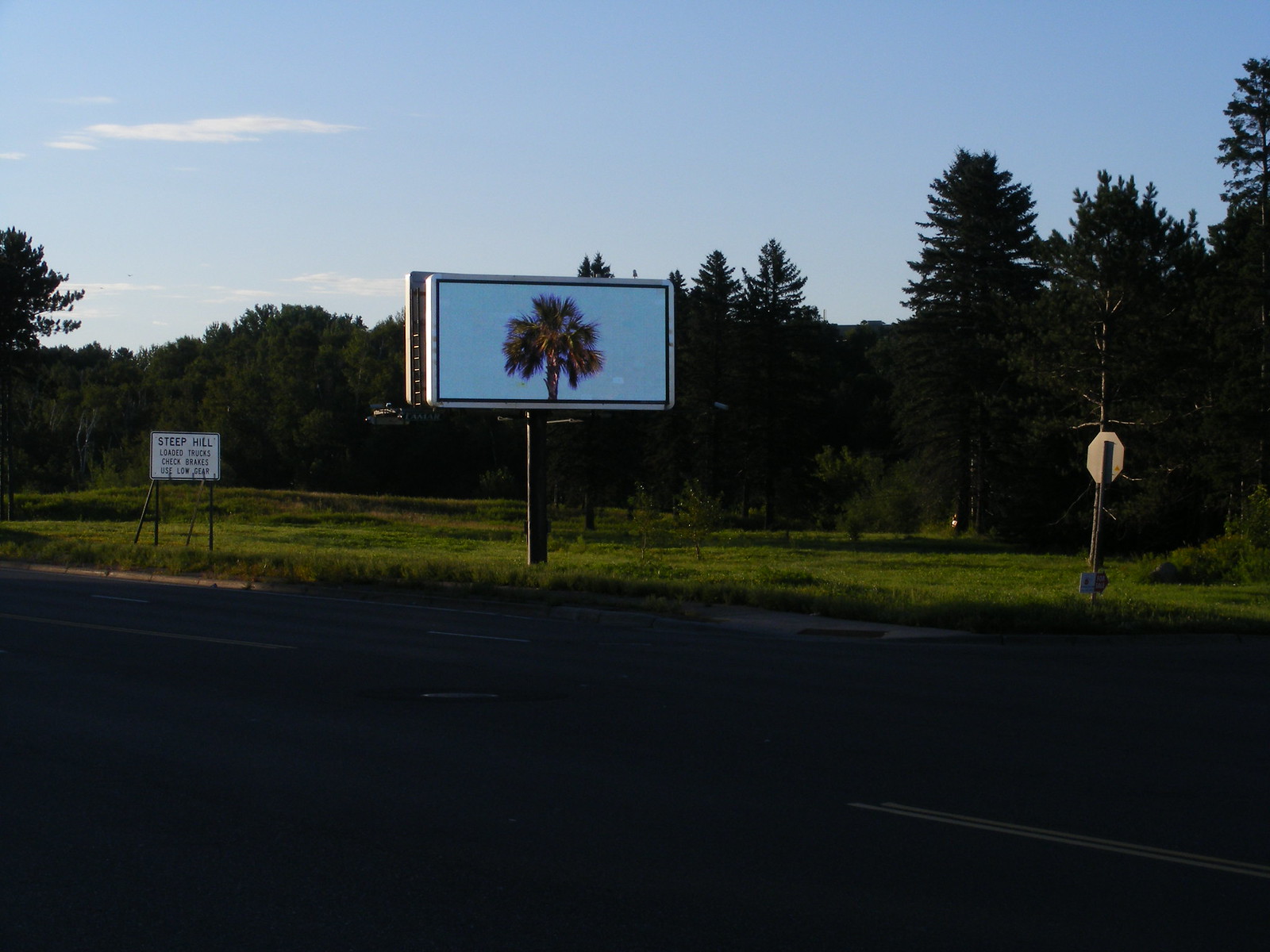This color photograph depicts a multi-lane highway with four or five lanes, stretching out under a nearly cloudless blue sky. The highway, marked by dark asphalt, is paralleled by a short strip of well-manicured, light green grass. In the background, a tree line comprises tall trees interspersed with bushes and hedges, all in varying shades of green.

Prominently featured in the middle of the image is a billboard mounted on a single cylindrical black post. The billboard displays an LED screen showing a blue sky with the top of a palm tree and its fronds. To the right of the image sits a stop sign. On the left, a white road sign with black text reads, "Steep Hill, Loaded Trucks, Check Brakes, Use Low Gear." The photograph is devoid of cars, people, and animals, emphasizing the serene, undisturbed nature of the scene.